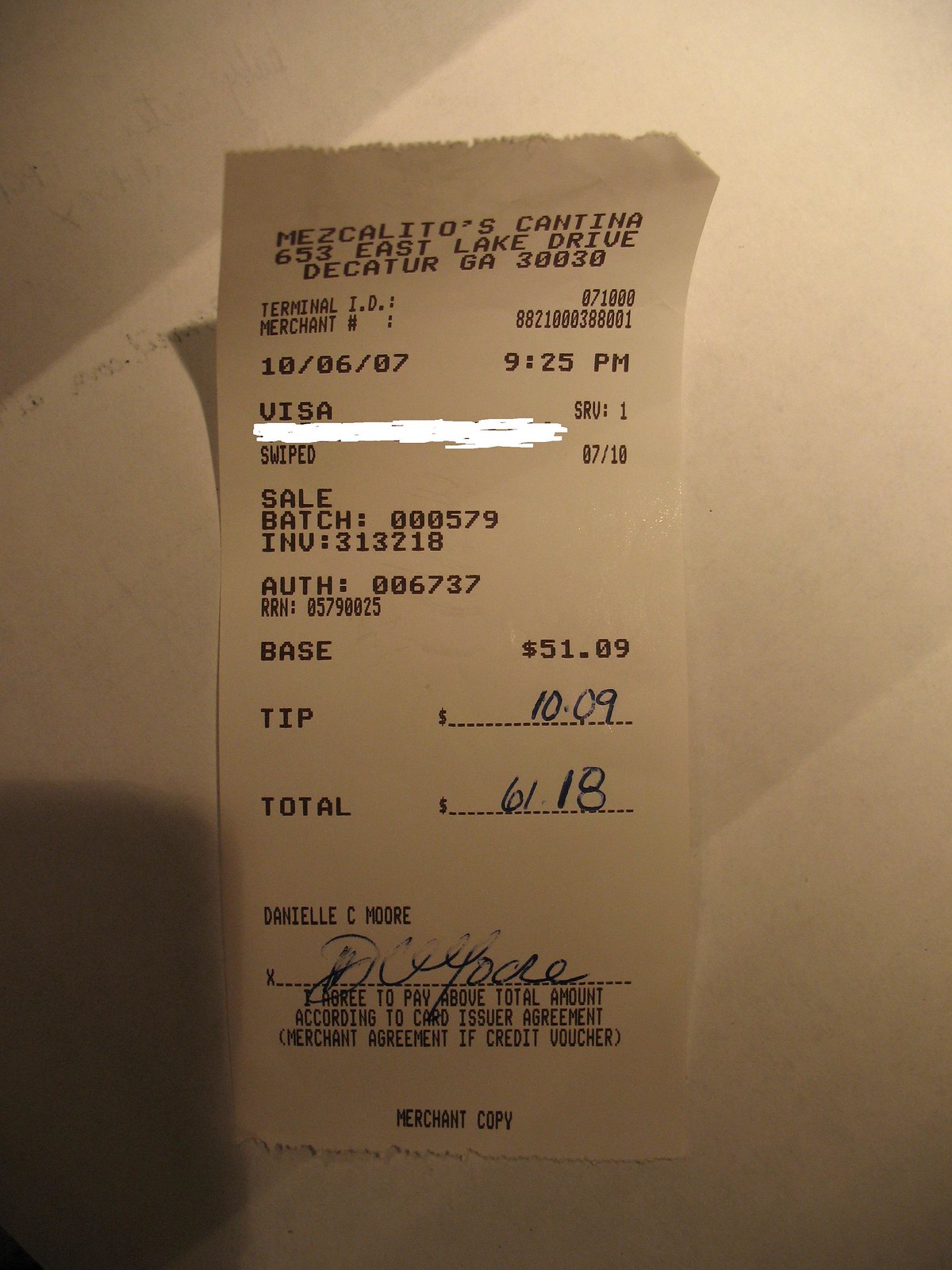This image features a receipt from Mezcalito's Cantina, located at 653 East Lake Drive, Decatur, Georgia, 30030. The receipt, predominantly white with a light gray tint, displays the date "10-06-07" and the time "9:25 PM" in the upper section. The credit card information is blurred out with a white stripe for privacy. The transaction details list a subtotal of $51.09, a tip of $10.09, both written in blue ink, culminating in a total of $61.18, with the total amount also in blue ink. Below these figures is the name "Danielle Seymour" and an accompanying signature. The surroundings of the receipt are light gray, with a pronounced shadow in the bottom left corner, giving the image depth and dimension.